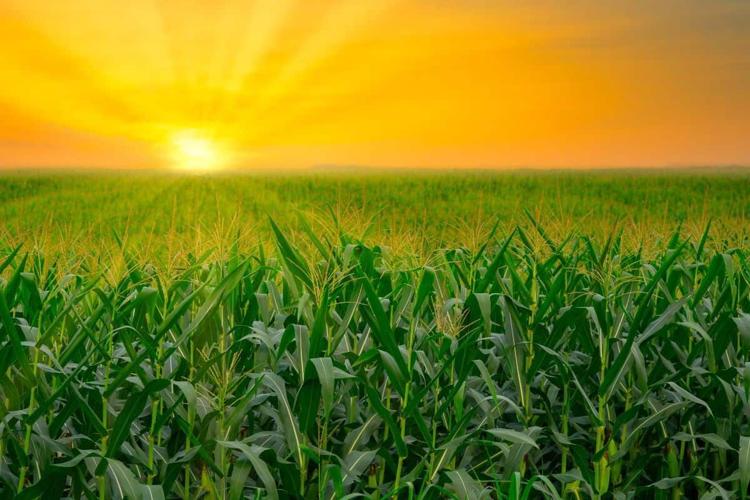An outdoor color photograph captures a vast, lush cornfield during either sunrise or sunset. The green, healthy corn stalks stretch out endlessly toward the horizon, where the sun's brilliant golden-yellow rays pierce through the sky, bathing the scene in a warm glow. The sky transitions from deep pinks near the horizon to vivid oranges and yellows, creating a stunning backdrop. The corn, though not yet fully grown, shows early signs of development, with tassels and partially formed cobs visible among the robust stalks. Sunbeams extend from the lower left of the image, casting a luminous yellow hue on the top of the corn, highlighting the tranquil beauty of this expansive agricultural landscape.